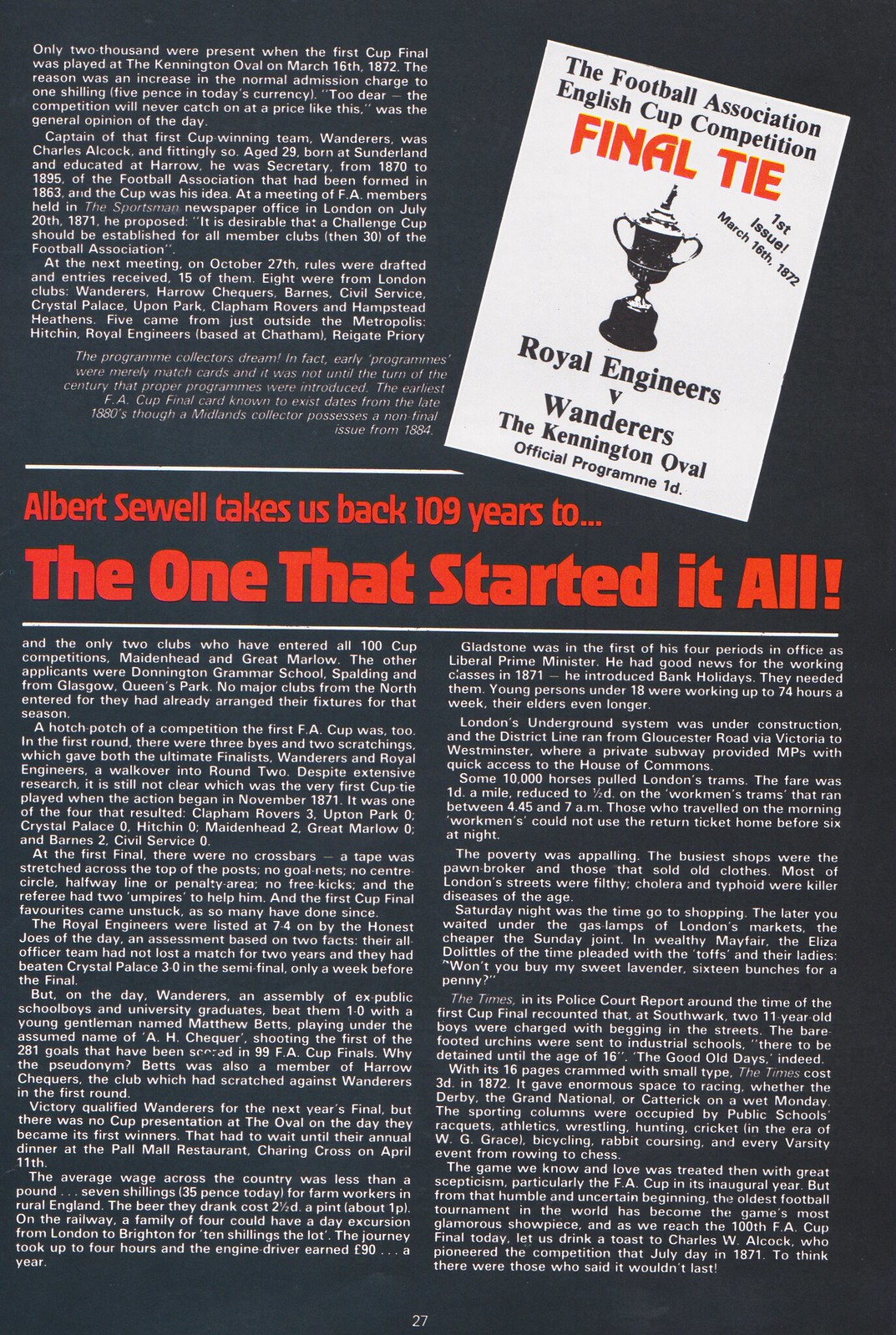The page is predominantly dark grey with a subtle gradient, almost black, and is from a magazine, specifically page 27. Dominating the upper part of the page, in the center, bold red text reads: "Albert Sewell takes us back 109 years to... THE ONE THAT STARTED IT ALL!" Below this heading, there is a white rectangular area occupying the upper right-hand corner with black and orange text. At the top, it displays, "The Football Association English Cup Competition" in black, followed by "Final Tie" in larger orange letters. Directly under this, it states, "First Issue, March 16, 1872" in black. The centerpiece of this white section is an image of a trophy, with text beneath it reading, "Royal Engineers v. Wanderers, the Kennington Oval Official Program 1D."

To the left of this white area and extending down the page, there's a detailed article recounting historical details of the event. The article describes the inaugural cup final match held at the Kennington Oval on March 16, 1872, highlighting the scarcity of attendance due to the elevated admission charge at the time. It delves into the background of Charles Alcock, captain of the winning team, Wanderers, and his pivotal role in proposing the establishment of the challenge cup, a concept he advocated during a Football Association meeting in 1871.

This advertisement doubles as a nostalgic retelling and a sales pitch, emphasizing the uniqueness and historical significance of the program, making it a prized collector’s item for soccer history enthusiasts.